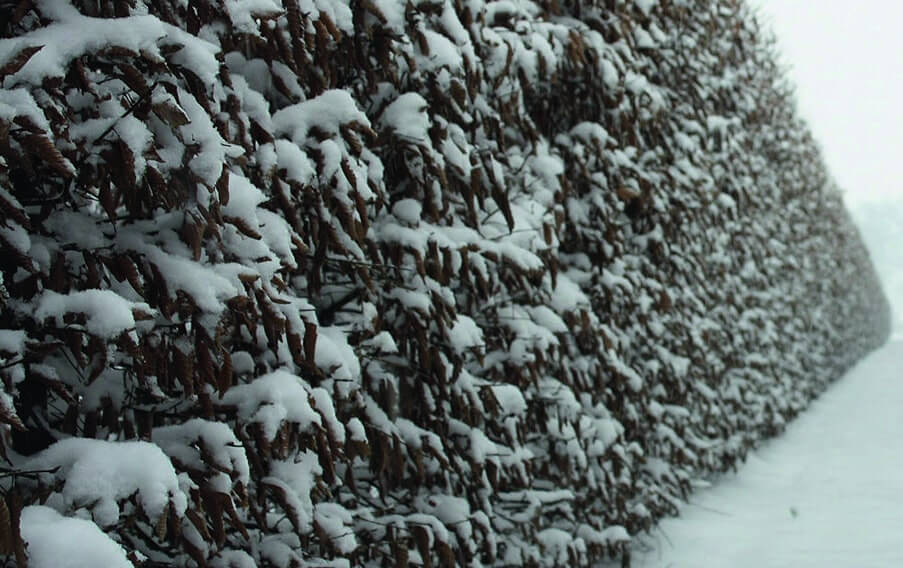This photo captures a close-up perspective of a hedge in a snowy outdoor scene. The hedge, heavily laden with thick piles of fresh snow, extends from the foreground on the left, where each branch and leaf is clearly visible, towards the right, where it becomes increasingly blurry, creating a depth effect. The leaves, some brown and curled, are weighed down by the snow, almost obscuring them entirely in places. On the ground to the bottom right, a snow-covered walkway is visible, adding to the wintry atmosphere. The hazy gray and white sky in the top right corner hints at ongoing snowfall, completing this serene, snowy landscape.